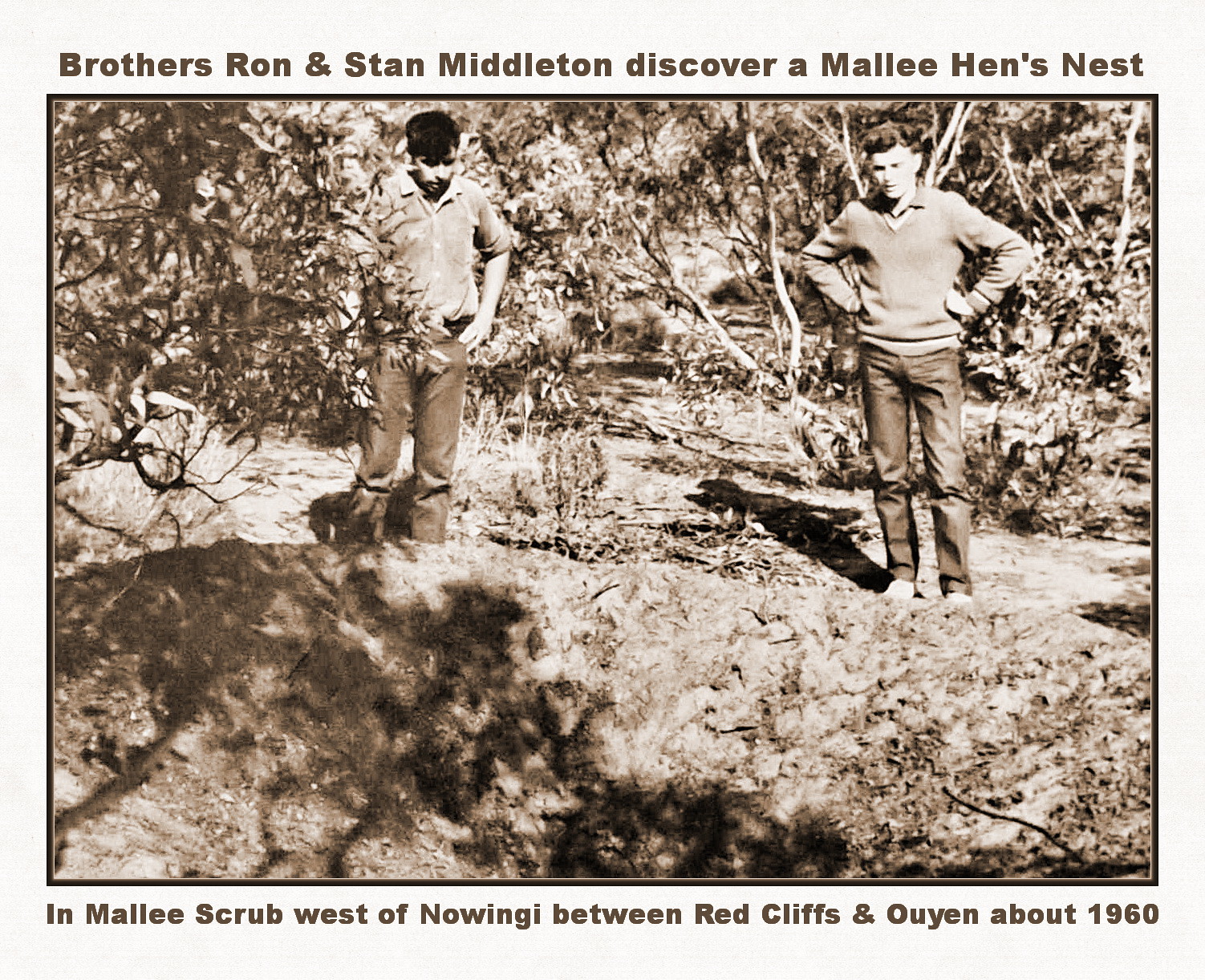A sepia-toned photograph captures two brothers, Ron and Stan Middleton, outdoors in the wilderness circa 1960. The scene shows them standing in front of a dirt pile or ditch, scrutinizing it closely. Ron, on the left, with black hair, wears jeans and a long-sleeved shirt with the sleeves rolled up. He has his hands in his pockets, looking down at the ditch. Stan, on the right, with blonde hair, has his hands on his hips, glancing towards the camera. The background features trees and grass, enhancing the rustic setting. The photograph is framed with a narrow brown frame and a wider white frame. In brown lettering on the white portion across the top, it reads, "Brothers Ron and Stan Middleton discover a Mallee hen's nest." At the bottom, the text continues, "In Mallee scrub west of Nowingi, between Red Cliffs and Oyen, about 1960."